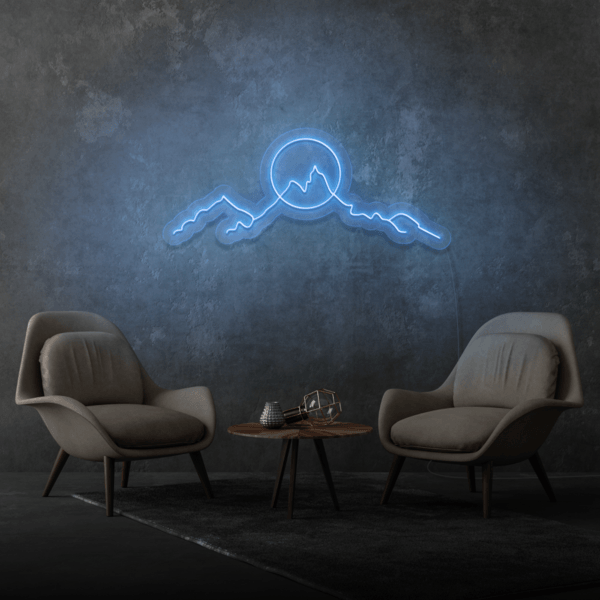The image, which is square-shaped and predominantly gray, depicts an indoor room with a stone wall as the backdrop. The wall, constructed of blocks of stone with light gray patches, occupies the upper three-fourths of the frame. Central to the wall is a piece of blue neon artwork, showcasing a mountain range with a circle—representing a sun or moon—atop the highest peak. Below the neon sign, there are two matching gray chairs with low backs and wooden legs, designed to face each other slightly, providing a cozy setup for conversation. These chairs feature gray cushions for both the seat and backrest. Positioned between the chairs is a small, three-legged round table, which holds a light bulb encased in a metal cage and a small silver cup. Extending from the lower right corner toward the left is a gray rug that complements the room’s color scheme.